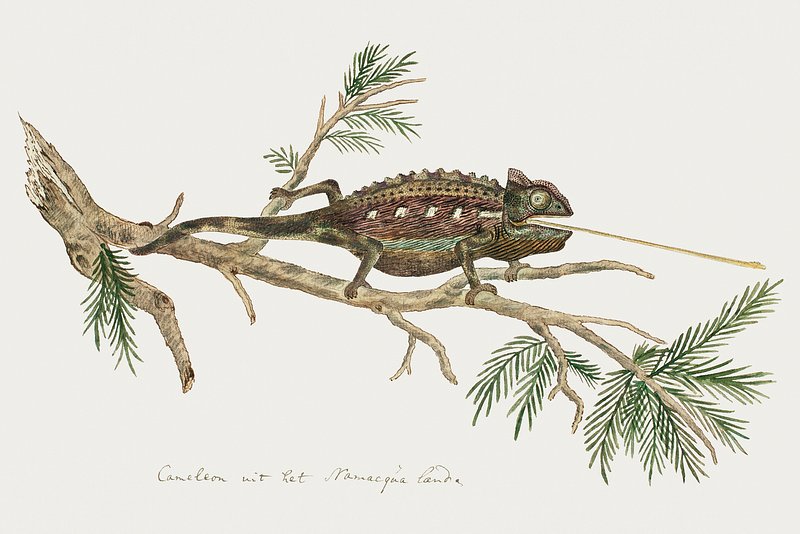The image is a detailed, colored drawing of a chameleon on an evergreen tree branch. The chameleon, which is styled in an abstract and artistic manner, features a flattened, oval-shaped body, particularly noticeable in the stomach area. Its body is a mix of brown, green, burgundy, and speckled gold, with shades of red, yellow, and blue hinting at its variegated coloring. The chameleon’s extended tongue, perhaps one-third the length of its entire body including the tail, protrudes as if it is attempting to catch an insect, though none is depicted. The creature’s limbs are wrapped around the branch, which splits into several sections with sparse, faint leaves. The branch supports the weighty tail entwining below. There's writing at the bottom of the image in cursive, partially decipherable as “chameleon,” followed by indistinct text that might be in a foreign language, hinting that this might be a scientific or botanical study drawing.